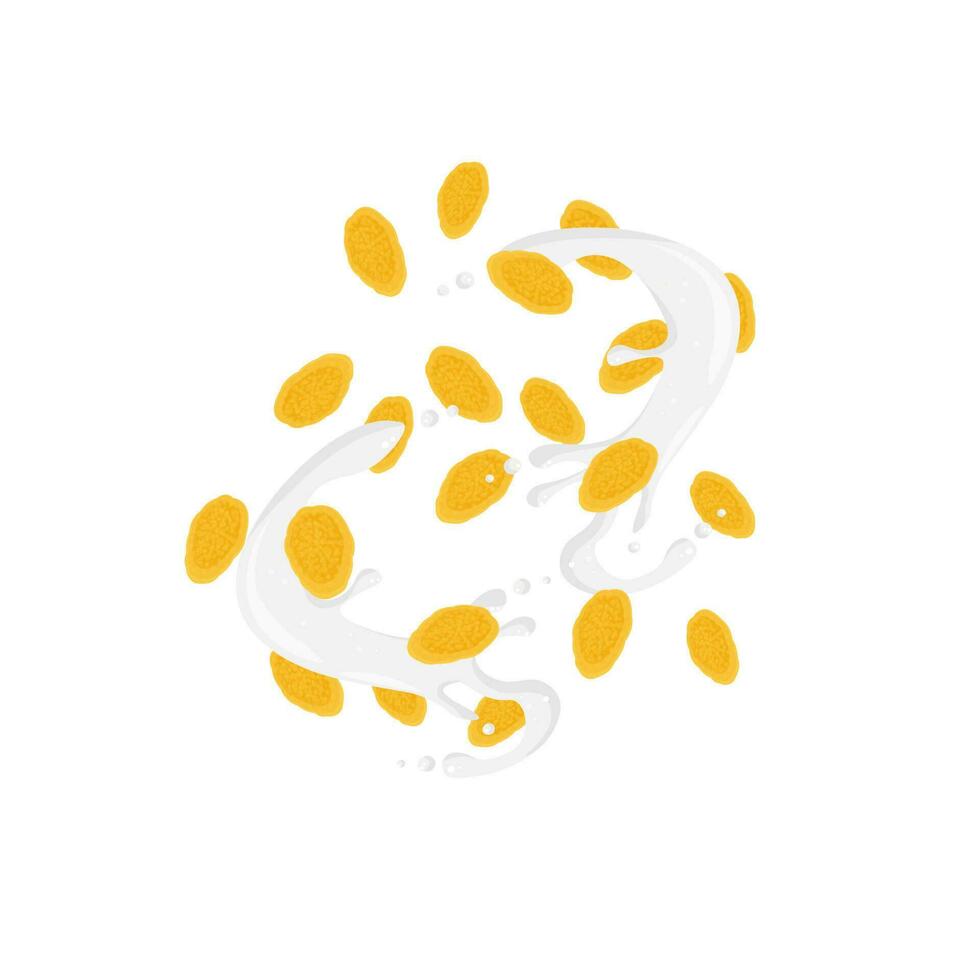The image is an artist's abstract portrayal featuring golden-colored seeds or crispy cereal ovals scattered across a white, swirling, and twisting background. These golden ovals, which can be compared to cornflakes or lemon slices, are dispersed throughout the scene without overlapping. The backdrop consists of subtle, creamy white liquid splatters and swirls, adding depth to the otherwise plain white canvas. The interplay between the crispy, golden pieces and the delicate, whipped cream-like splatters creates a mesmerizing and intricate visual experience.